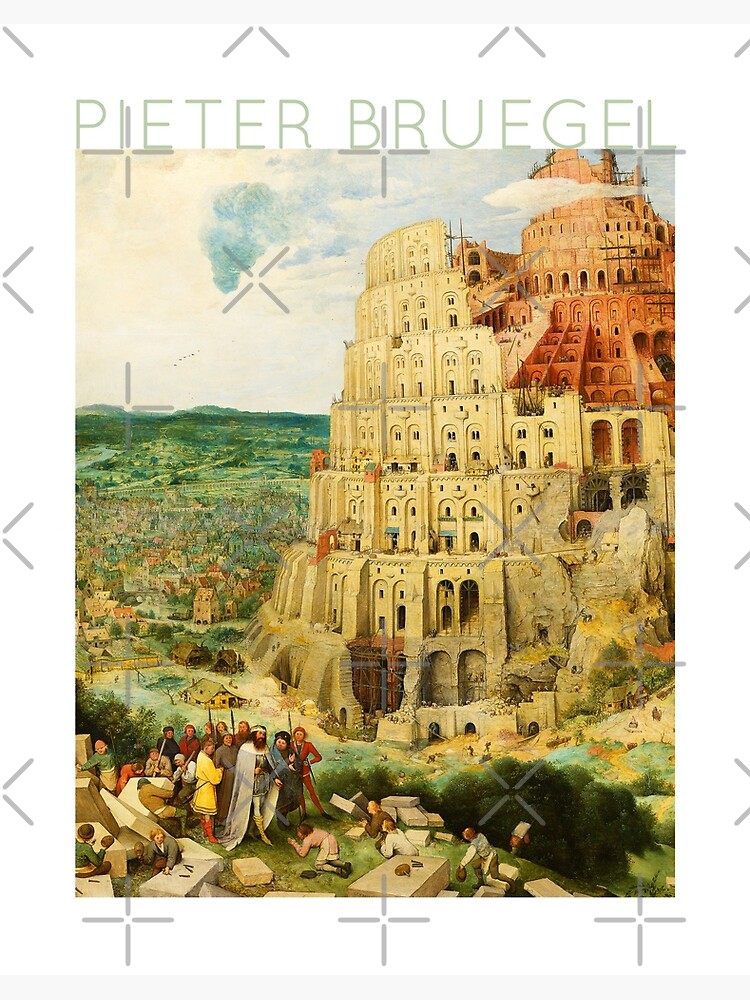This artwork, attributed to Peter Bruegel, depicts the construction of a monumental multi-tiered tower, reminiscent of the Tower of Babel. The tower, primarily composed of light tan or beige stone with a bronze or darker brown hue in the center, stands unfinished at the top. The scene features a bustling ancient town where groups of bearded men are engaged in various tasks such as chiseling and forming stone blocks. A man dressed in a white robe, possibly a king, stands surrounded by others, overseeing the progress. The distant horizon reveals verdant rolling hills and stylized blue and gray clouds, with one cloud strategically placed in front of the tower to emphasize its towering height. The sky heightens the overall dramatic atmosphere of this historic setting. The image is marked with grey crosshairs and an X-shaped pattern, suggesting it might be a proof print.